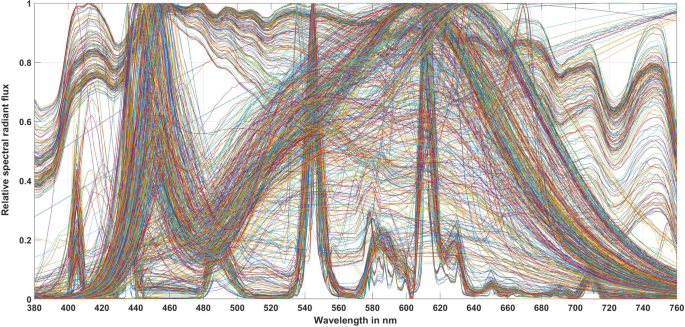This image is a horizontal rectangular graph displaying a relative spectral radiance flux. Along the bottom, the horizontal axis is labeled "Wavelength" and measures wavelengths in nanometers (nm) from 380 to 760. The vertical axis is marked with numbers, although the specific label is unclear. The graph features numerous colorful lines, resembling hair, in shades of red, orange, green, and more, indicating different readings or data sets. These lines undulate up and down across the graph, creating a dynamic and intricate pattern. While there appear to be letters interspersed among the lines, suggesting the presence of variables or annotations, the exact legend or key explaining these elements is not visible. Overall, the image presents a complex and highly detailed scientific representation of spectral data fluctuating over a range of wavelengths.